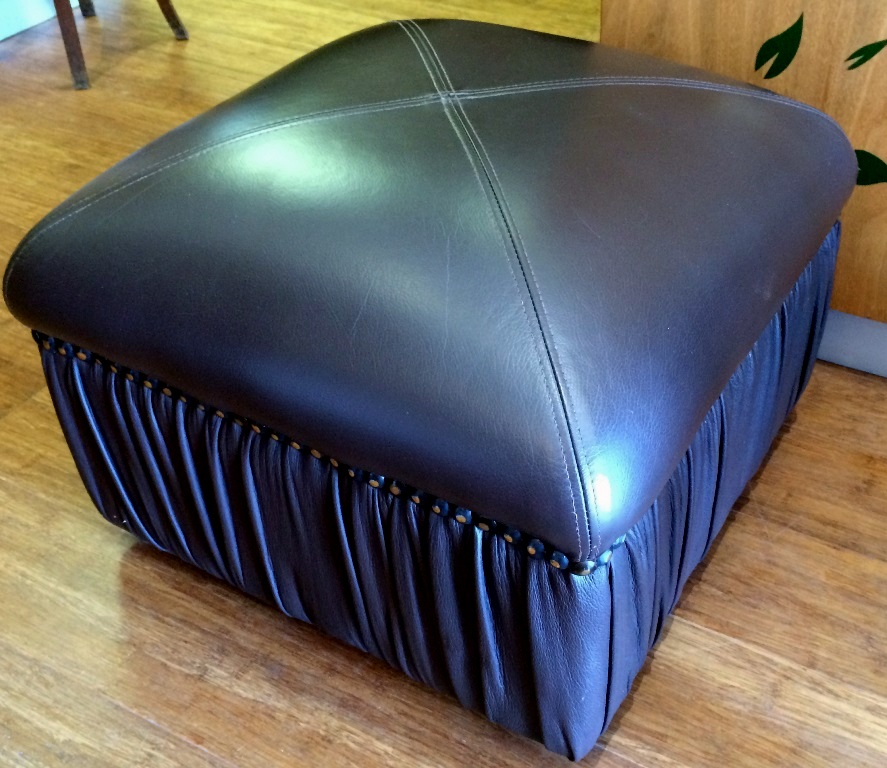In the image, there's a dark blue leather ottoman or footstool resting on a brown hardwood floor. The top of the ottoman is rounded with diagonal stitching forming a cross-hatch pattern, creating an X shape. Surrounding the top part are blue beads with gold dots in the center, secured with tacks all around its circumference. Below the beaded section, the leather is folded and bunched, extending almost to the floor, resembling a skirt. The room features a brown wooden table or countertop with an etched design of green leaves in the background. Additionally, a wooden chair with three visible legs can be seen in the top right corner of the image. The overall setting suggests an indoor environment.